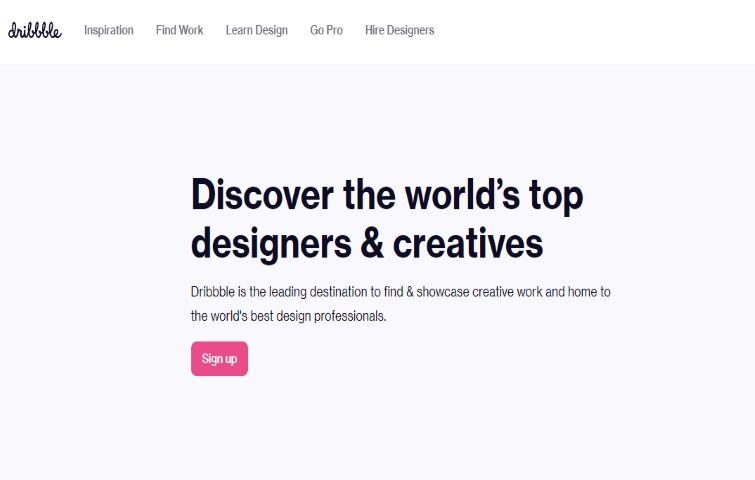This image is a screenshot from the Dribbble website, known for its three B's in the name. The header is adorned with several navigation options in white script, including "Inspiration," "Find Work," "Learn Design," and "Go Pro." These options are anchored by a light gray background along with a call to action, "Hire Designers," also in light gray text. Dominating the page is a large, light gray box featuring a prominent headline in big, bold black letters, stating, "Discover the World's Top Designers and Creatives." Beneath this header, a subtext explains, "Dribbble is the leading destination to find and showcase creative work and home to the world's best design professionals." This section is complemented by a small, hot pink box with the text "Sign Up" in white writing, inviting users to engage. The header options do not feature dropdown menus, and there are no icons or symbols accompanying the Dribbble branding other than its distinct script logo. The layout emphasizes the platform's primary focus on connecting and highlighting creative professionals.